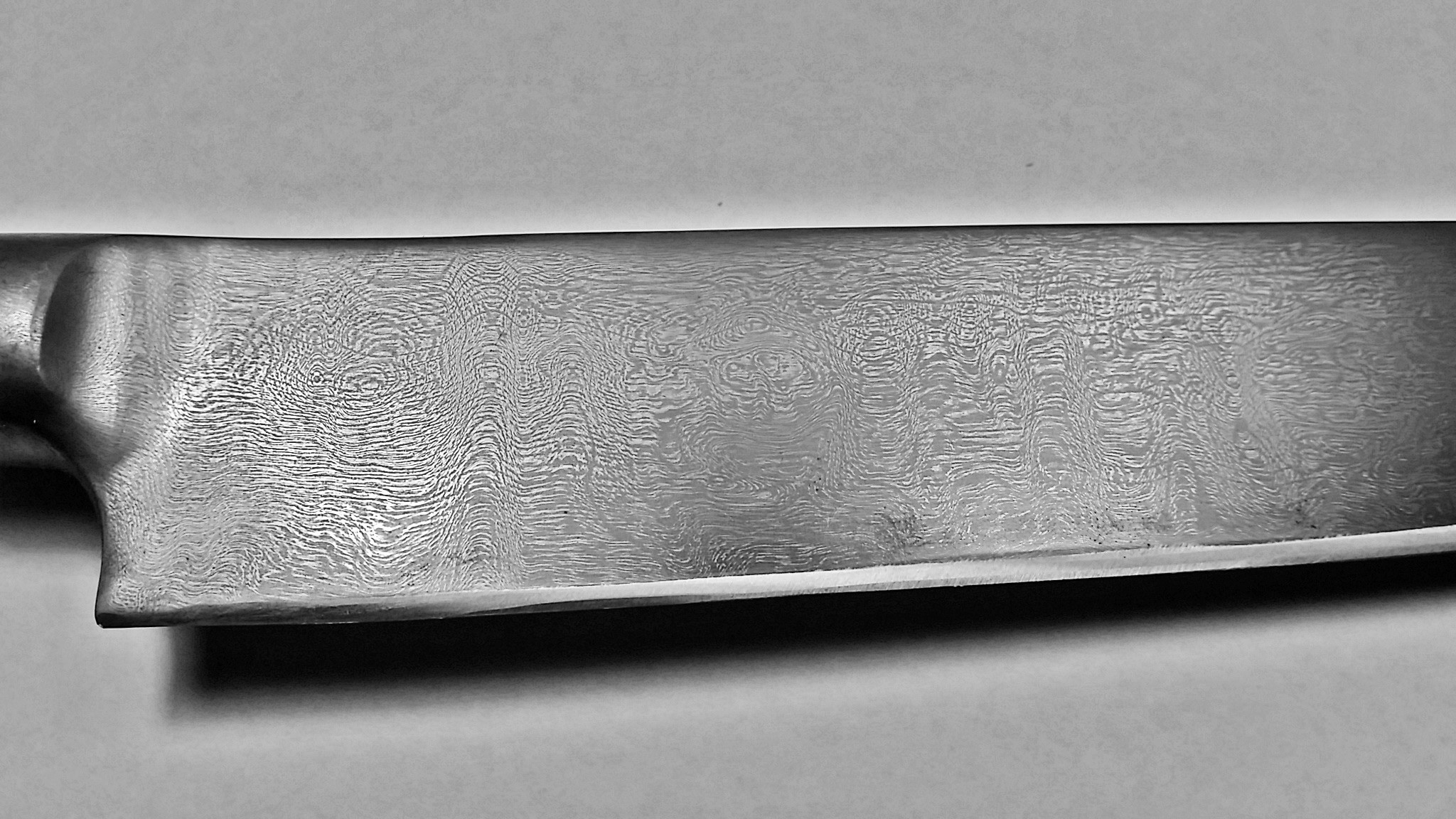The image is a horizontally long, rectangular photograph with a gray background, depicting a knife that is prominently placed in the center. The knife appears shiny silver with a grainy, ripple-like pattern on its blade, suggesting handcrafted quality. Only part of the handle is visible, and it is primarily the same silver color as the blade, though slightly darker. There is a dark gray, almost black shadow beneath the knife, emphasizing its presence against the flat surface. The knife exhibits a polished sheen, potentially indicating it has been digitally enhanced, making it stand out against the uniform backdrop. The overall impression is of a meticulously crafted and possibly edited image showcasing the knife.